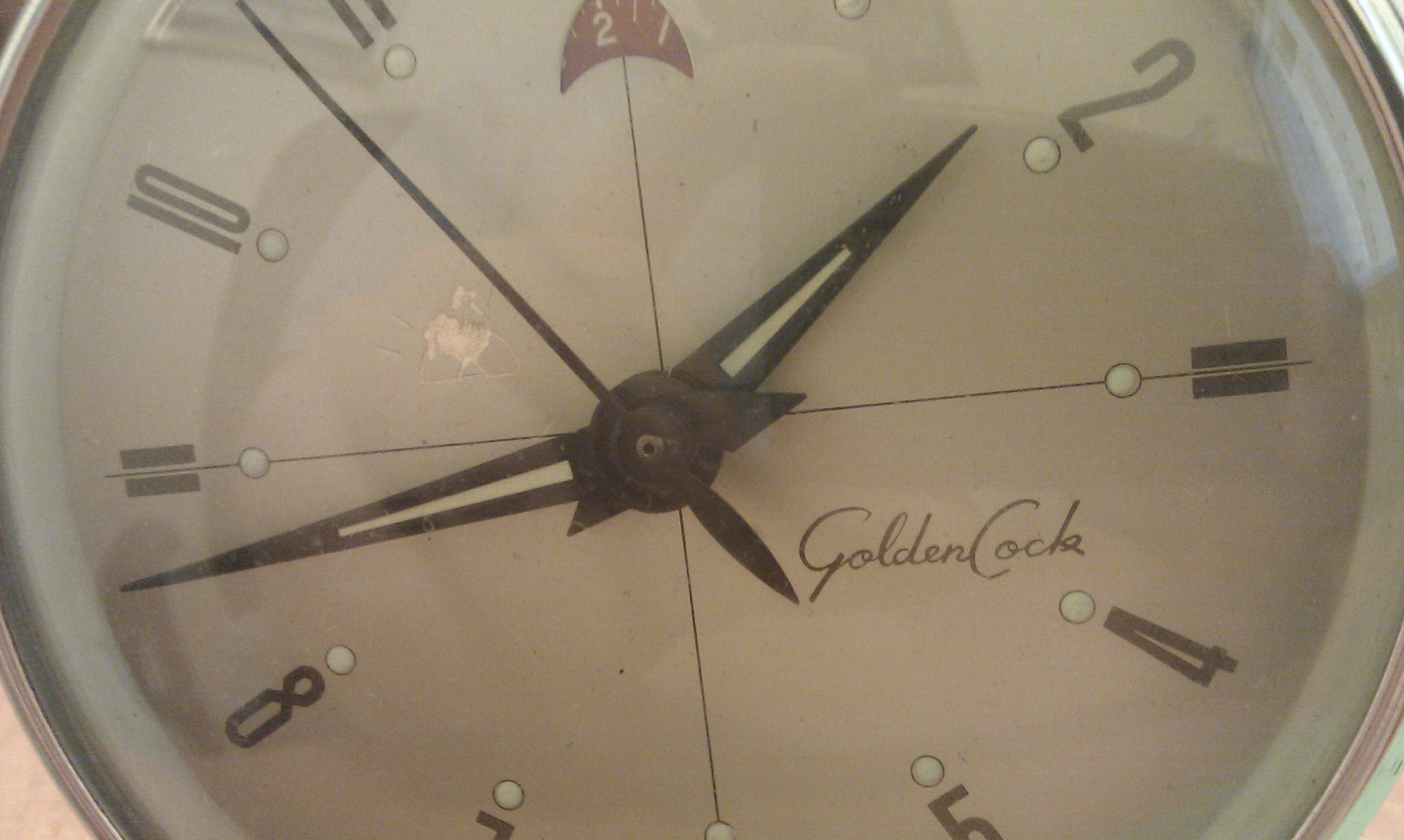This image captures an extreme close-up of a clock face, focusing only on its central portion, such that the edges of the clock are not visible. It reveals that the clock face is white with black hour markers, and the hour, minute, and second hands are made of a black material, either metallic or plastic. The visible numbers include two, four, five, seven, eight, ten, and part of eleven, while the positions of three and nine are marked by black dashes. The clock indicates a time close to 2:45. Notably, on the right side of the face, there is a script font logo that reads "Golden Cock," which likely denotes the brand or maker of the clock.